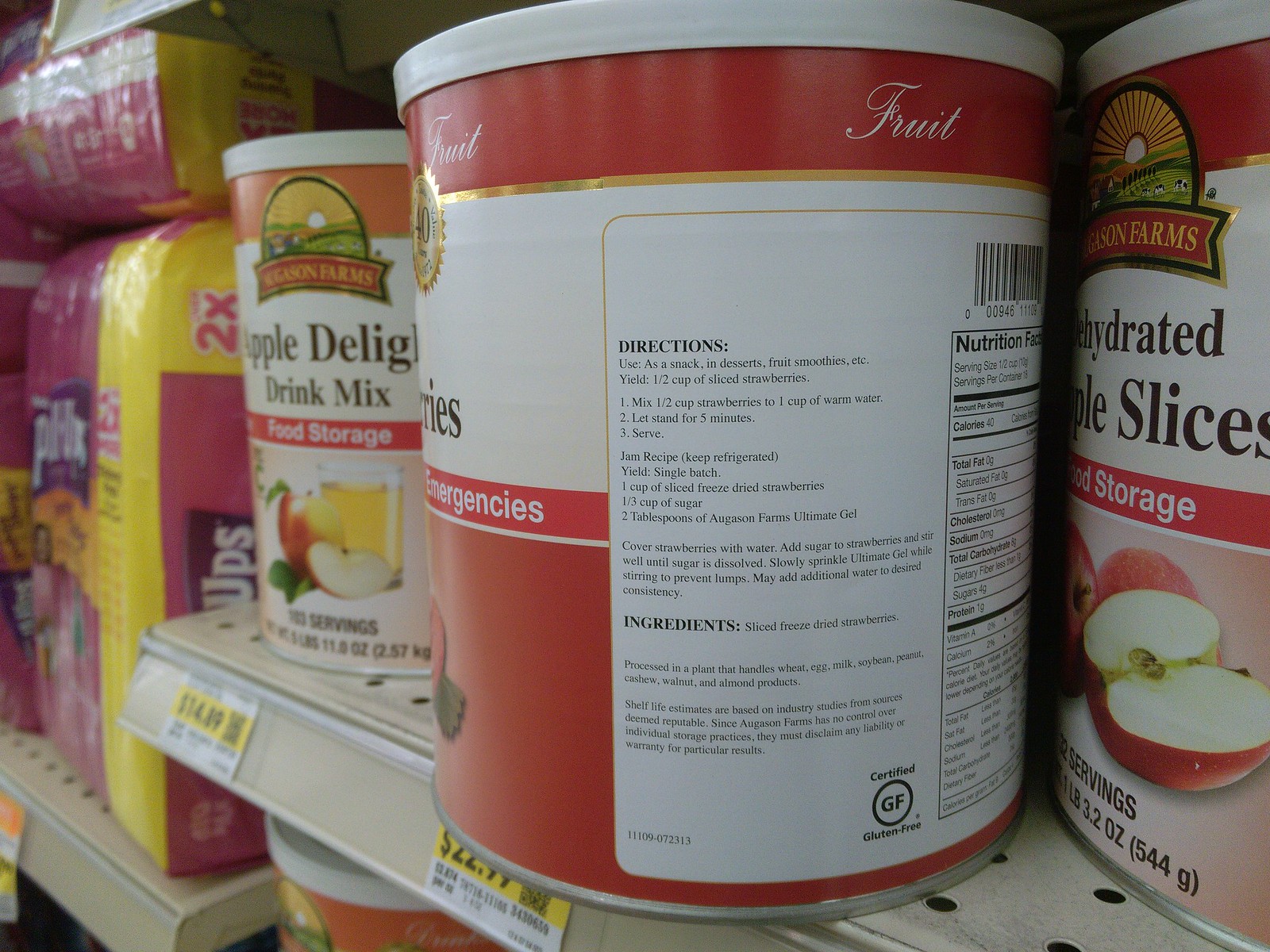The image depicts a well-organized shelf inside a grocery store, featuring an array of emergency food supplies prominently placed in red and white, 12-ounce cylindrical containers. These containers advertise products such as "Apple Delight Drink Mix" and "Dehydrated Apple Slices," with detailed labels showcasing nutritional facts and mixing directions, albeit in very tiny, hard-to-read writing. The labels also feature farm imagery with a glass of juice and an apple. Adjacent to these emergency food items, one can observe packages of diapers or pull-ups on the left side, distinguishable by their pink and yellow-colored packaging and the word "Pull-Ups" displayed prominently. Price tags, characterized by a white background with a yellow rectangular highlight, are visible throughout the image with prices displayed in black, showing amounts such as $14.89 and $22.99. The beige shelf enhances the organized display, making the items and their respective price points clearly visible, despite some difficulty in reading smaller text details.